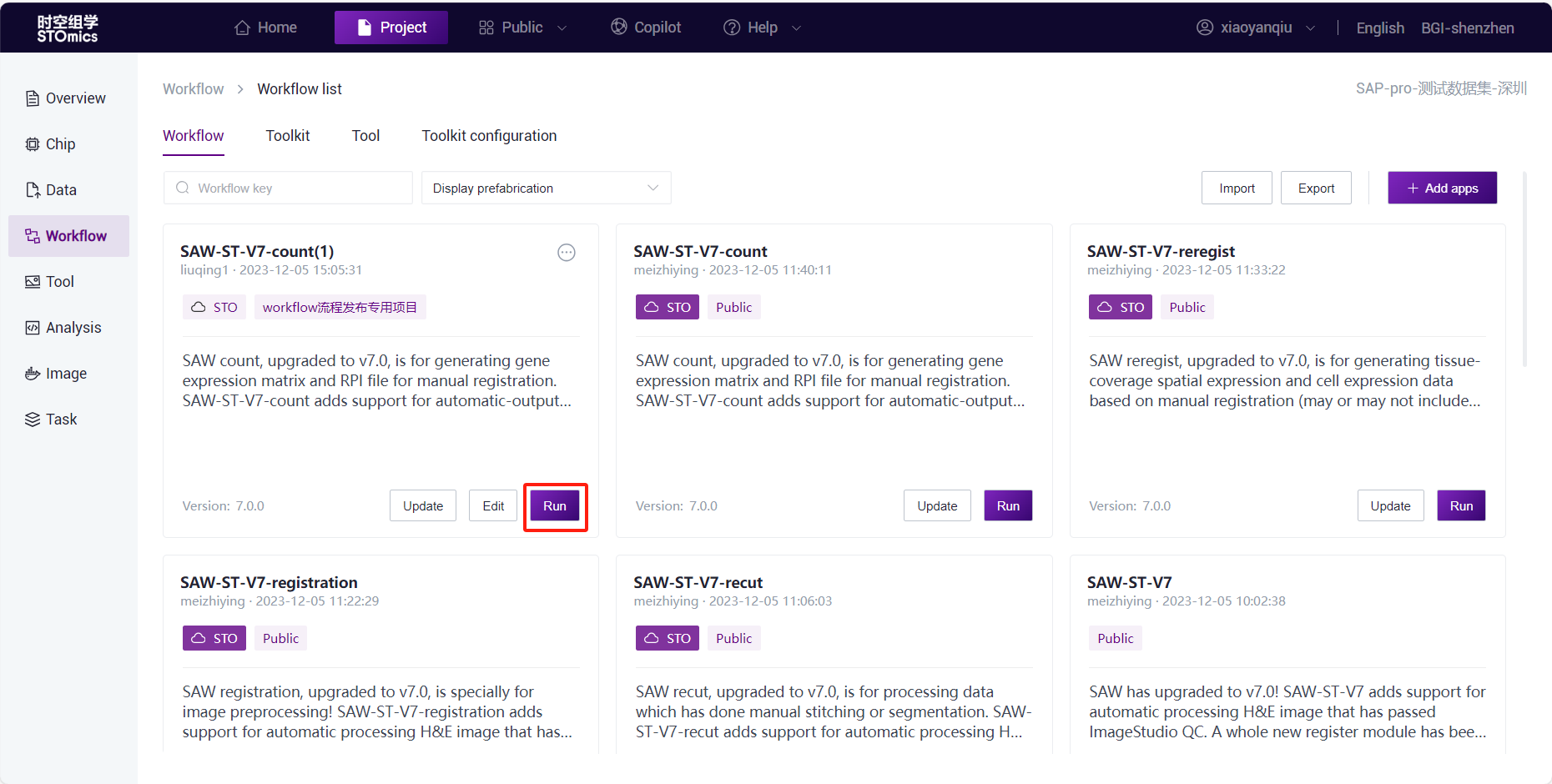The image is a detailed screenshot of a utility page potentially utilized by IT professionals. The top border of the interface is black, with the upper left corner displaying the label "STO" in capital letters followed by "mics" in lowercase, and above it, there are characters that appear to be in Chinese or Japanese.

To the right of this text is a horizontal menu bar. The menu items are labeled in the following order: "HOME," "PROJECTS," "PUBLIC," "CO-PILOT," and "HELP." Notably, "PROJECTS" is highlighted, appearing in white text against a purple background, signifying that the page displayed belongs to the "PROJECTS" section. The other menu items are written in grey text on the black background. 

On the far right of the menu bar, the word "ENGLISH" is visible, followed by text obscured and unreadable, possibly indicating a language setting. Further to the right is what looks to be a username, starting with "X-I-A-Y-A-N" and possibly continuing with "Q-U." Beneath this, the text "SAP PRO" in capital letters is displayed, hinting that the software is related to SAP. To the right, more untranslated Chinese characters can be seen. 

The main body of the page has a white background and is segmented into six distinct sections. Each section has a header in bold black font starting with "SAW-ST-V7," followed by different extensions unique to each segment. Purple rectangles are adjacent to most section headers.

On the left side of the page is a narrow sidebar with a very light blue background. This sidebar contains a vertical menu listing the following items from top to bottom: "overview," "chip," "data," "workflow," "tool," "analysis," "image," and "task." This arrangement hints at a systematic workflow or navigation pattern for various functionalities within the application.